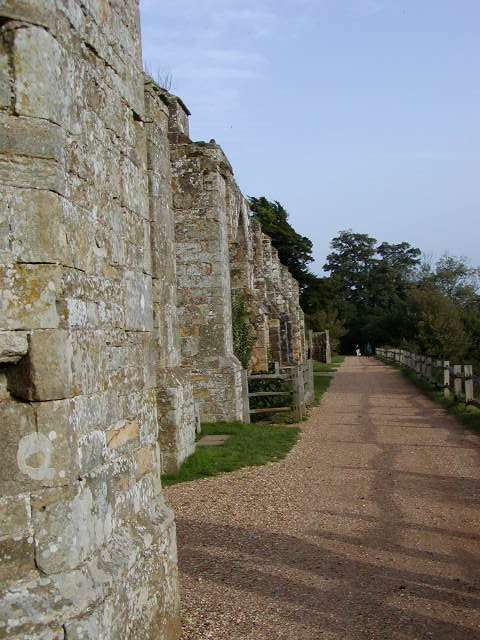The photograph captures a serene archaeological site with a gravelly, reddish-brown dirt path running through the center. To the left, towering granite stone walls reminiscent of an ancient castle stretch down the road, their imposing presence evoking a sense of history. These meticulously stacked stones form a significant, albeit weathered, structure possibly indicating a former stronghold or significant building from antiquity. On the right side of the path, a short wooden fence casts shadows on the ground under the bright sun, adding a rustic charm to the scene. The well-maintained path is flanked by patches of green grass, enhancing its walkable appeal. The background fades into a dense forest with dark green trees under a clear, cloudless blue sky, creating a vivid contrast with the ancient stones and modern upkeep. This balanced composition of historical remnants and natural beauty offers a picturesque glimpse into the past.